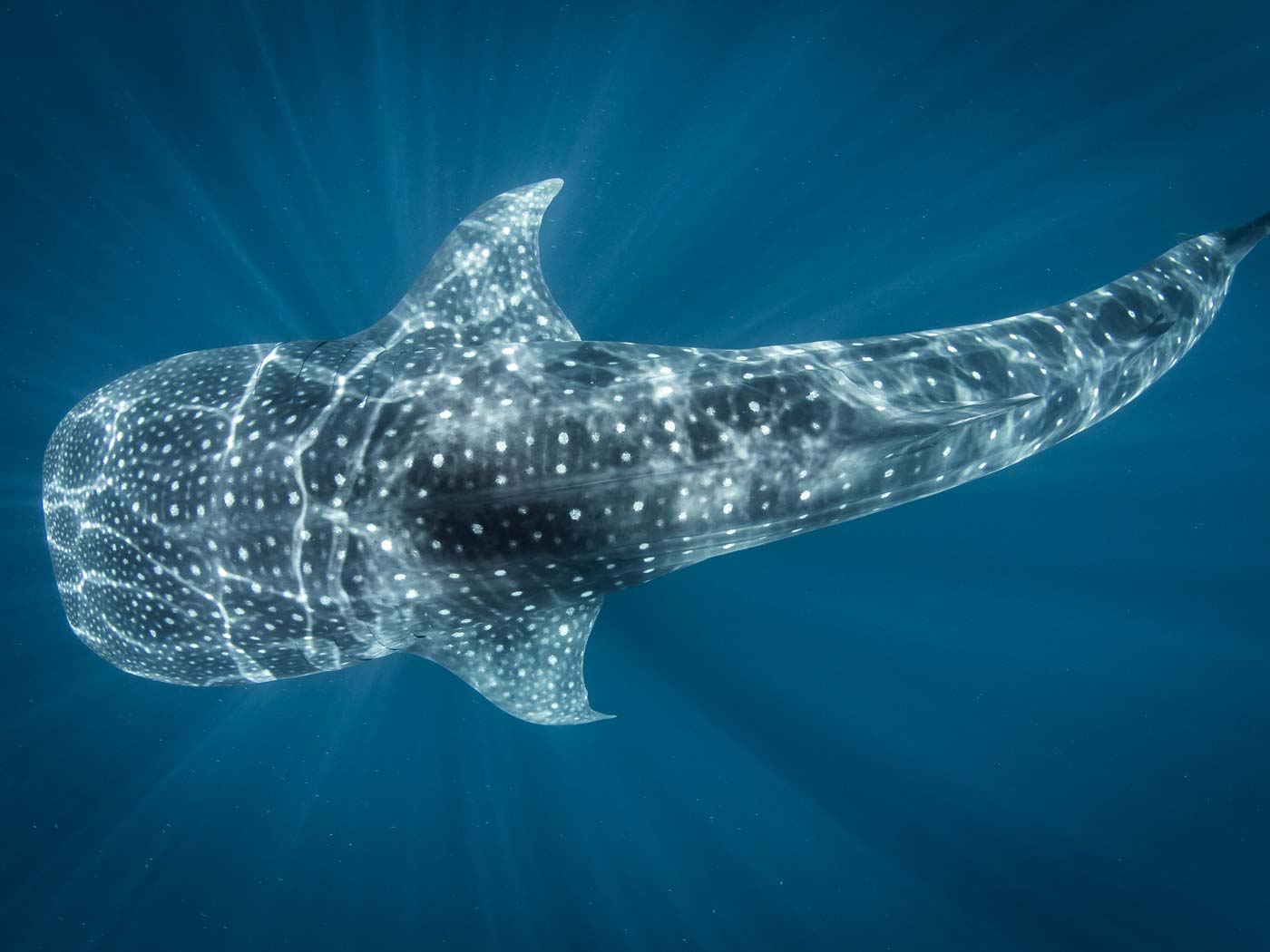The overhead photograph captures a large marine creature, most likely a shark, swimming from right to left through blue waters. The animal fills the majority of the frame with its dark gray, round-shaped head positioned on the left. Its body is adorned with bright white spots, more concentrated near the head and fins. The creature features distinct gill slits along its sides, indicating it is not a whale but a type of fish. Two triangular fins flank its body, and it has a long tail fin that curves upward, suggesting motion. The blue water beneath it transitions from darker at the edges to lighter near the creature, with light rays appearing to shine up from beneath, adding an ethereal glow to the scene.